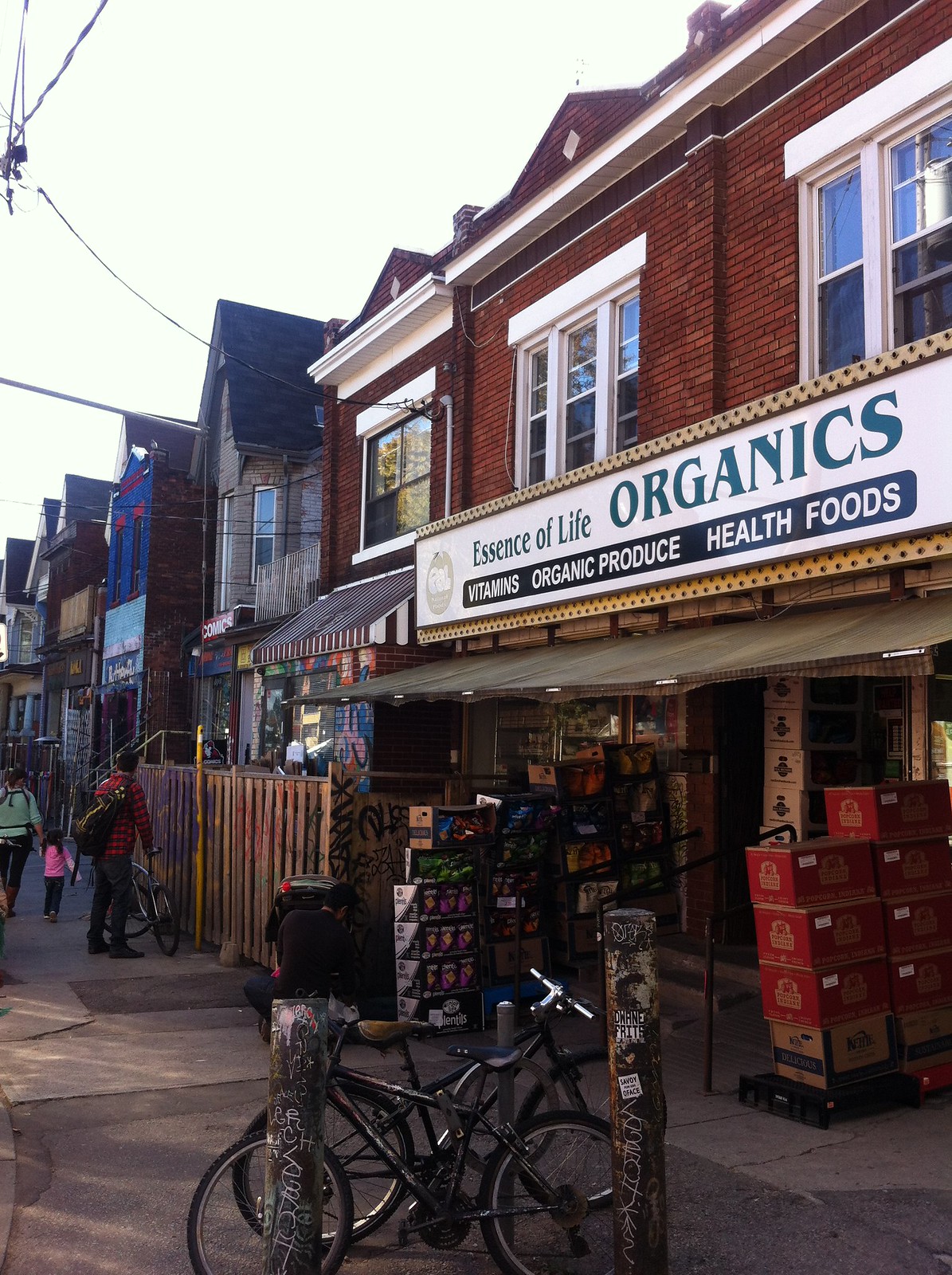In this sunny and bright photograph, a bustling street corner captures a vibrant scene in front of the Essence of Life Organics store. The store's distinct white rectangular sign boasts blue lettering that reads "Essence of Life Organics" with a black strip underneath detailing "Vitamins, Organic Produce, Health Foods" in white text. The storefront, built from horizontally-laid brick, features large windows suggesting potential apartments or additional business spaces above it.

In the foreground, two poles with unreadable graffiti support two bicycles that lean against them. Directly in front of the store, numerous boxes filled with varied products, likely produce and health items, are on display. A man crouches near these boxes, possibly handling them or interacting with another person close by.

Further along the strip to the right, an individual wearing a red plaid shirt, jeans, and loafers—with a brown backpack and a bicycle—stands in front of another store. To the left, a woman in a blue or green top, dark pants, and boots holds the hand of a little girl dressed in a pink top, jeans, and tennis shoes. The scene is lively with the interplay of these characters while the sunlight beams off the building windows, accentuating the photo's clear, weather-free day.